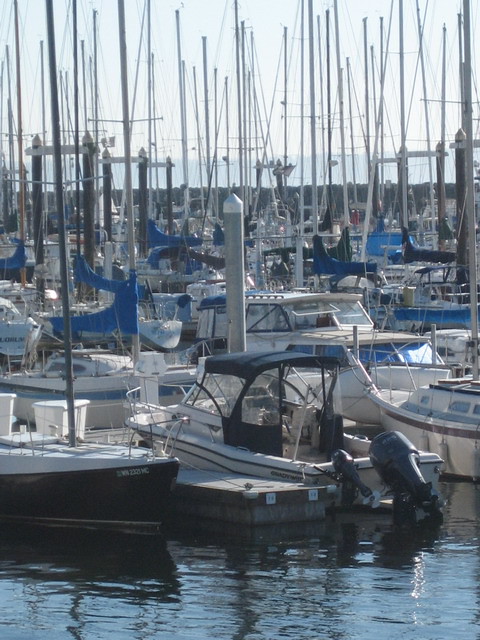This color photograph captures a bustling marina filled with dozens, possibly hundreds, of moored boats and yachts, predominantly white with some blue striping and detailing. The scene is dominated by the tall, vertical masts of the sailboats that extend high into an overcast, light blue-gray sky, indicating a lack of direct sunlight. At the very bottom of the image, a small portion of the calm, reflective water is visible, showing dark blue to brownish hues with a few indistinct black reflections. The background transitions seamlessly into more boats, dense and closely packed, with a hint of a horizon that may feature a seawall or distant trees. The docks in the photograph are made of wood, and none of the boats have their sails open. Some of the nearest boats appear to have black motors at their sterns, faintly reflected in the water. The marina seems devoid of people, emphasizing the serene yet crowded arrangement of the vessels against the muted sky.